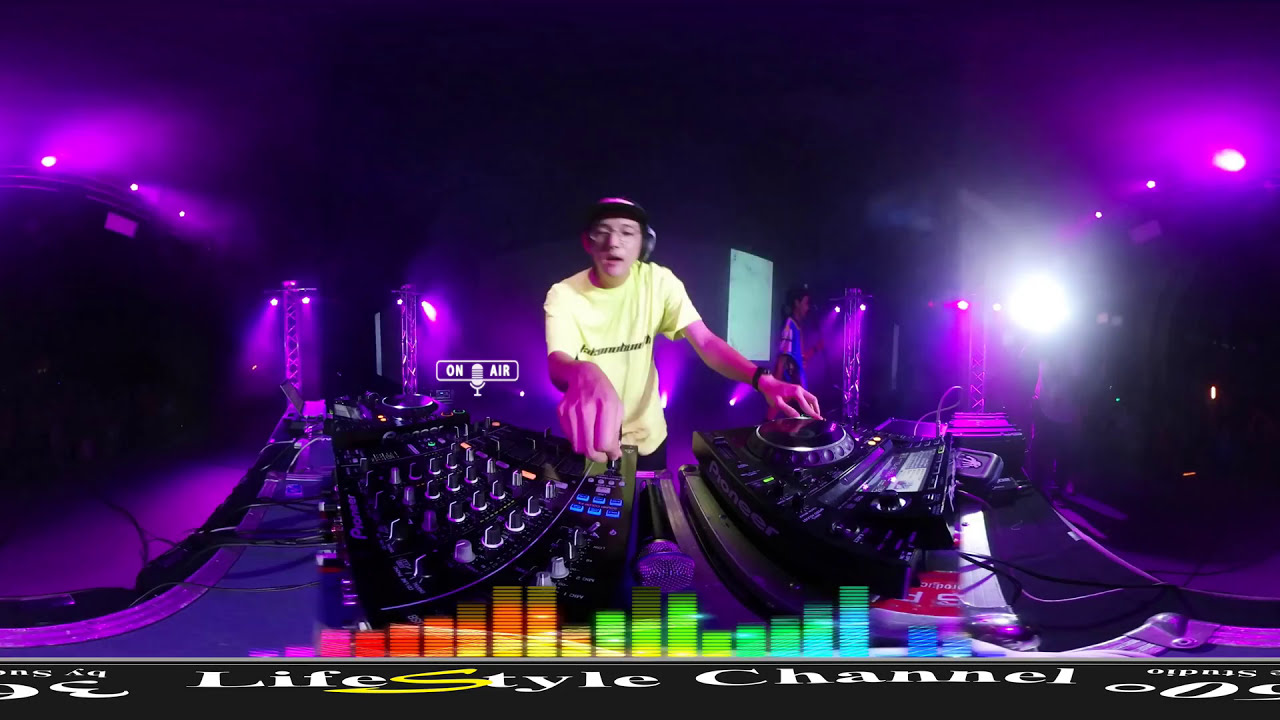The image captures a dynamic scene of a DJ deeply immersed in his performance at a DJ board. The DJ, likely a young Caucasian man, is centered in the frame and wearing a bright pale yellow or white shirt that potentially features the word "Amsterdam" in black text. He is also seen wearing glasses and possibly a hat, with earphones on and his mouth slightly open, indicating focus and engagement in his craft. His left hand is interacting with a circular black turntable, while his right hand manipulates an array of buttons and levers, incorporating a grid of knobs and controls. The entire scene is bathed in a wash of purple and pinkish lights, with a few bright white lights accentuating the setup, creating a vibrant and energetic atmosphere. The panoramic, 360-degree angle adds a unique distortion to the image, making the proportions appear rounded and skewed. At the bottom of the image, a dark gray bar features the text "Lifestyle Channel" in white letters, with the 'S' highlighted in yellow. Above this, a rainbow-colored sound bar enhances the visual appeal. The scene is further enlivened by an "On Air" sign illuminated in the mid-section, alongside potential glimpses of a second individual in the background, enhancing the sense of a lively, electrifying environment.